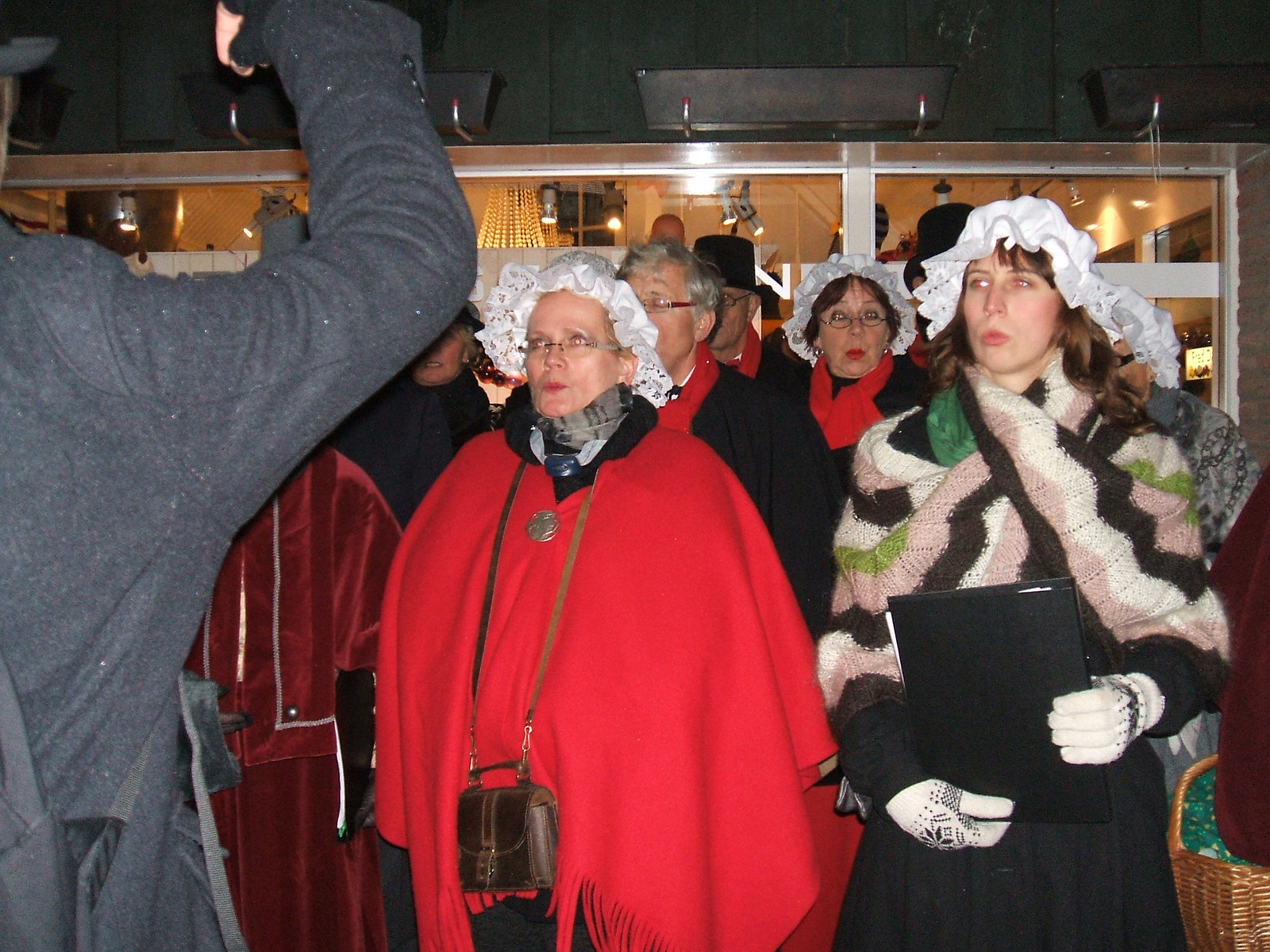The image depicts a group of Christmas carolers gathered indoors, possibly in front of a well-lit storefront. The majority of the group consists of women wearing traditional caroler attire, including white frilled bonnets adorned with eyelets and lace. The central figure is a prominent woman in a large, red poncho, with a leather bag slung over her neck. To her immediate right is another woman in a crocheted or knitted shawl featuring pink, white, and blue stripes. She is also wearing white gloves with a fair isle print and holds a black bound book. To the far right of the scene stands a woman in a thick, pink sweater-jacket with brown hair partially covered by a white headdress. A man in a dark-colored coat stands on the left, visible from the back, with his arm raised as though conducting the choir. The carolers, a mix of both older men and women, many adorned with red scarves, appear to be singing festively, evoking a sense of holiday spirit.